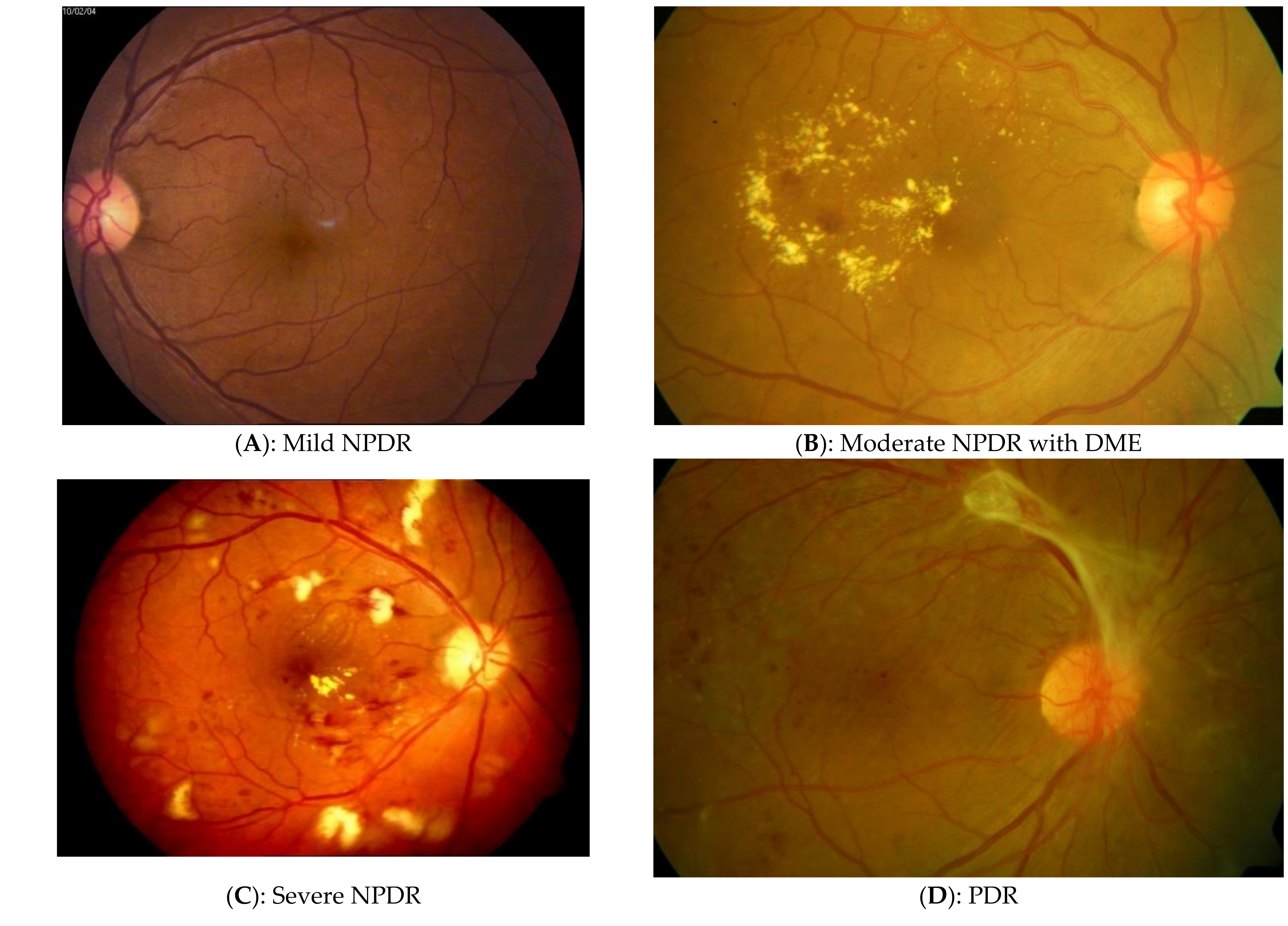This detailed infographic features four close-up images showing different stages of an eyeball condition known as NPDR and PDR. Each image is set against a black background and visually represents the progression of this medical condition. 

The first image, labeled "A. Mild NPDR," depicts a relatively healthier eyeball with a yellowish center and visible veins. It shows the initial phase where abnormalities are minimal. 

The second image, titled "B. Moderate NPDR with DME," portrays a more advanced stage, with a yellowish-red hue and intricate veins, indicating increased severity. DME likely stands for diabetic macular edema, suggesting additional complications.

The third image, captioned "C. Severe NPDR," features a highly red sphere with prominent white spots and dense red veins, illustrating significant progression and heightened abnormalities. 

Finally, the fourth image, "D. PDR," presents a closer view of the eyeball, further emphasizing the abnormal vein structures and possibly indicating proliferative diabetic retinopathy, a severe stage of the condition with extensive damage and new, abnormal blood vessel growth. Each image subtly highlights different features and irregularities to depict the disease's progression, making it an informative diagnostic tool or educational reference.